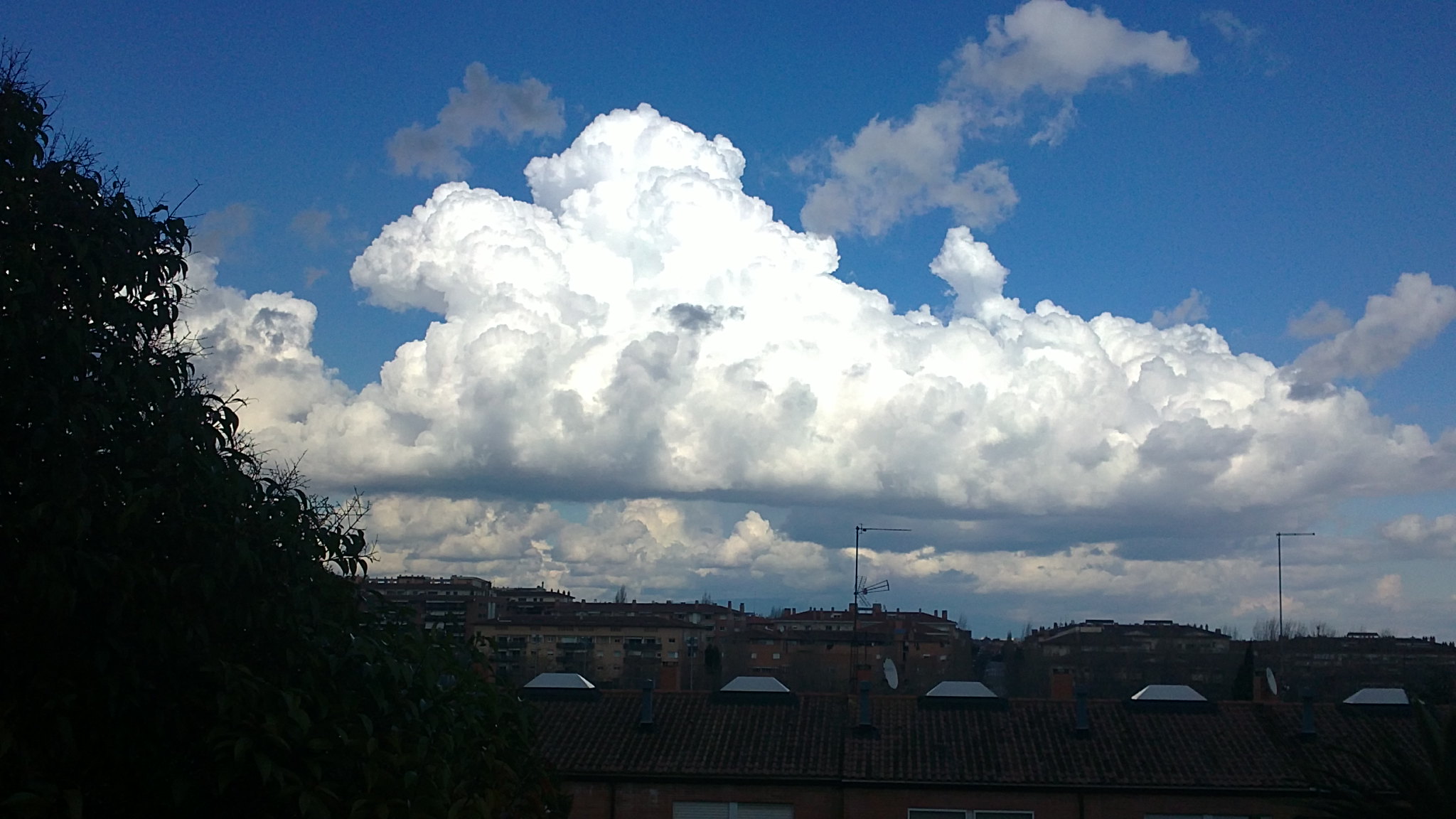This outdoor photograph captures a predominantly blue sky adorned with large, towering white clouds with grayish bases, which make up the majority of the image. The clouds are the primary focus, highlighting their dramatic presence against the clear blue sky. Below the cloudscape, the scene becomes darker and more challenging to discern, although some elements are distinguishable. On the left, there are shaded trees or large bushes. The bottom center reveals the tops of buildings, possibly apartments or businesses, featuring a brown roof equipped with five white, solid-colored vents. Further in the distance, more buildings are visible, and the skyline hosts several tall poles, likely antennas. The overall image offers a striking contrast between the illuminated sky and the shadowed elements below.